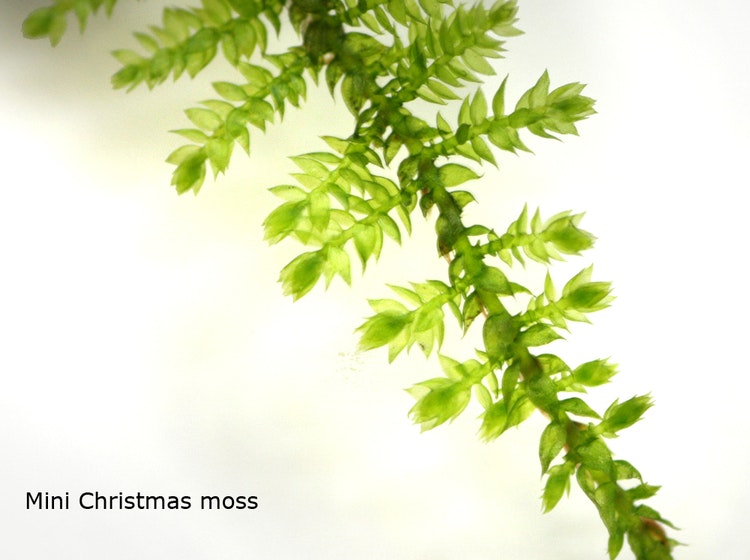The image presents a detailed close-up of mini Christmas moss, as indicated by black text in the bottom left corner. The background is predominantly white with a slight tan gradient towards the top, giving the moss an almost ethereal quality that seems to blend into the surroundings. The plant itself extends diagonally from the top left to the bottom right of the image, displaying its vibrant green hue that ranges in different shades. The plant structure resembles a miniature tree, where the base is narrower, and the branches—each with tiny, somewhat translucent leaves—become progressively smaller towards the bottom. The leaves appear semi-transparent, allowing light to filter through and enhance their delicate, almost glass-like quality, making the overall appearance very striking and unique.